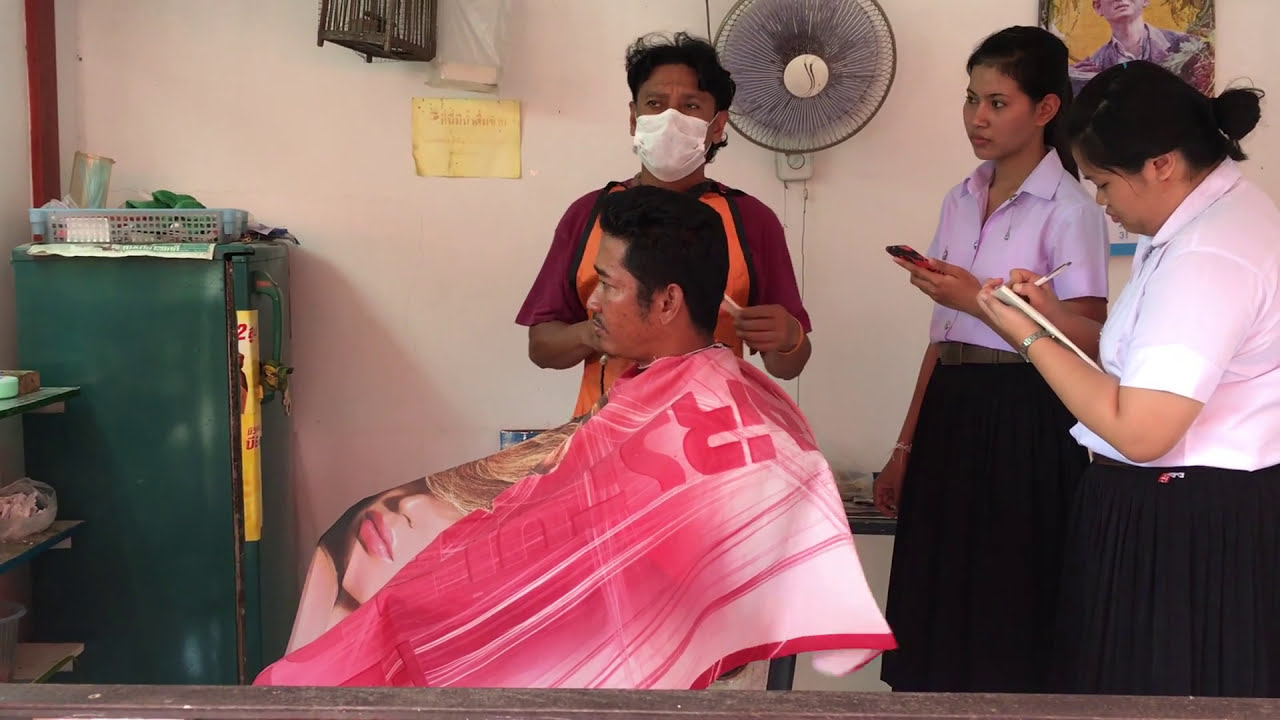The image depicts a scene inside a barbershop with four individuals who all appear to be of Hispanic or South Asian heritage. At the center, a man with dark, thick hair, styled in a short, puffed-up manner, is seated sideways in a barber's chair, facing the left. He has a mustache and a towel wrapped around his head. The man appears to be in the process of getting a haircut, as he is draped with a pink smock adorned with white lines, pink writing, and a striped border.

Behind the man is the barber, wearing a medical face mask, a maroon shirt, and an orange apron with a black border. Standing to his left are two females, each dressed in a light lavender short-sleeve collared shirt and a black skirt. One girl is holding a phone, possibly recording or taking notes, while the other appears to have a clipboard.

The background features a light beige wall with several items hanging on it, including an oscillating fan and various pictures. A green cabinet or refrigerator-like object is placed in front of the seated man to the right (but on the left side of the photograph). This green cabinet has something yellow on its surface and a light blue basket on top. Additionally, a shelving unit is visible beside the cabinet, holding various items such as green and light blue objects, and a semi-translucent plastic jug.

The room contains a broad palette of colors, including green, pink, purple, white, black, tan, yellow, orange, and red, indicating a lively and busy environment. Overall, the photograph captures an indoor setting populated with individuals engaged in typical barbershop activities.